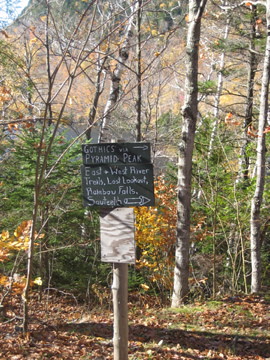The image showcases a densely forested area with various tree trunks, some of which appear barren and devoid of leaves, while smaller green trees or shrubs fill in the underbrush. The terrain itself is strewn with leaves, adding to the forest ambiance. Centrally positioned is a weathered tree supporting a sign with a black placard that's partially obscured but visibly bearing the names "Pyramid Peak" and "Gothics." The sign also includes directional arrows pointing towards several hiking trails such as "East and West River Trails," "Lost Lookout," and "Katsuba Falls Southeast." The arrows indicate the directions to these destinations, suggesting it's a guidepost for hikers navigating the forest trails.